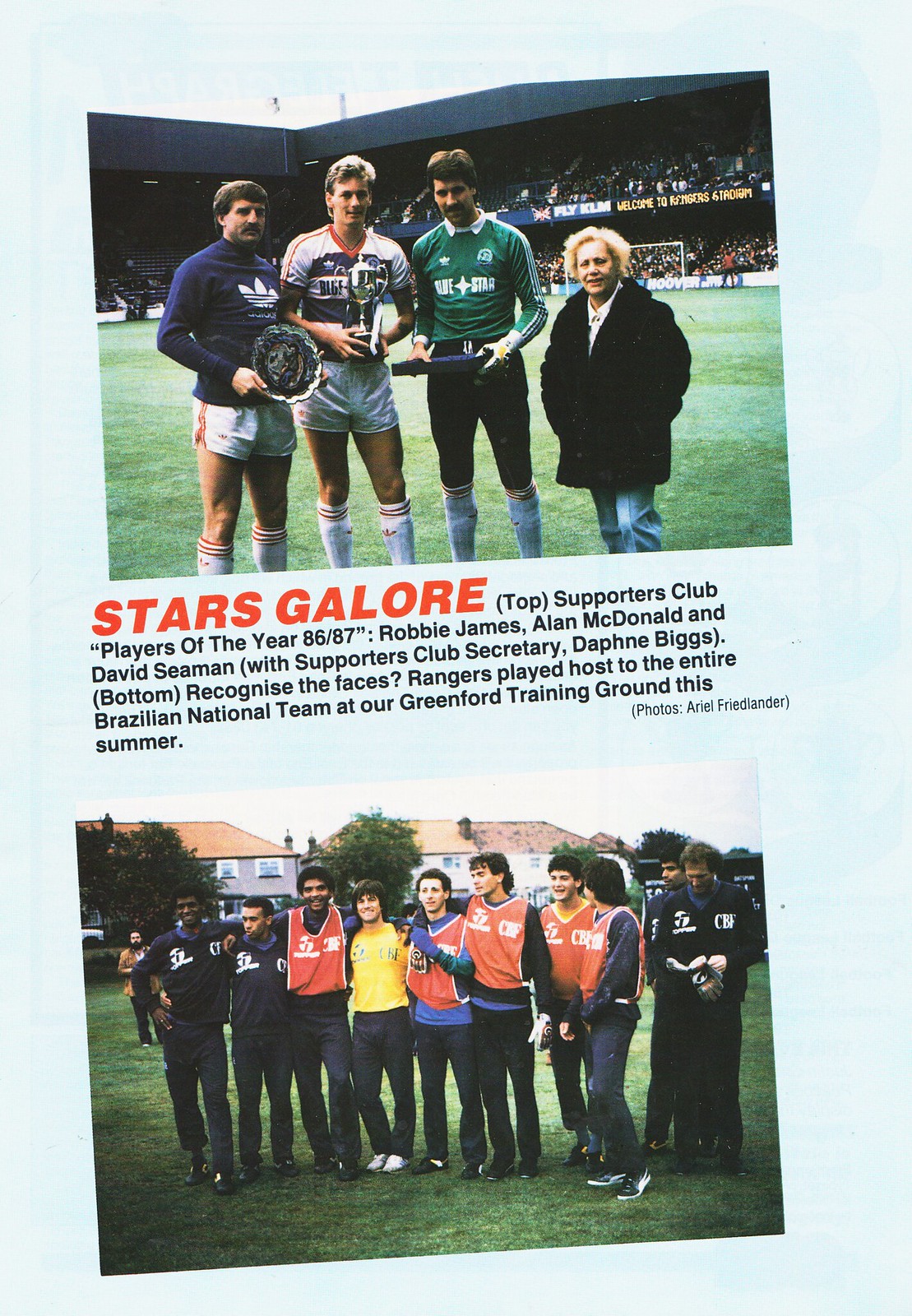This image is a scan from a sports magazine, featuring a light blue or gray background with two photographs angled upwards towards the upper right. The first photograph, positioned at the top, captures a celebratory moment on a soccer field. It features three soccer players, each holding a trophy, and wearing different colored jerseys, indicating they are from different teams. Standing beside them is an elderly woman with frizzy hair in a black coat. The stadium in the background is filled with spectators. Text beneath this photo reads, "Stars Galore, Supporters Club Players of the Year 1986-1987, Robbie Jennings, Alan McDonald, and David Seaman, with Supporters Club Secretary Daphne Biggs."

The second photograph, located at the bottom, is also tilted and presents about ten individuals posed on an outdoor field, possibly a training ground. They are wearing long pants and a mix of orange and black jerseys, suggesting they are members of a soccer team, dressed for cold weather. Houses can be seen in the background. The accompanying text states, "Recognize these faces, Rangers played host to the entire Brazilian national team at our Greenford training ground this summer." At the bottom of the page, there is a small credit that reads, "Photos by Ariel Freidlander."